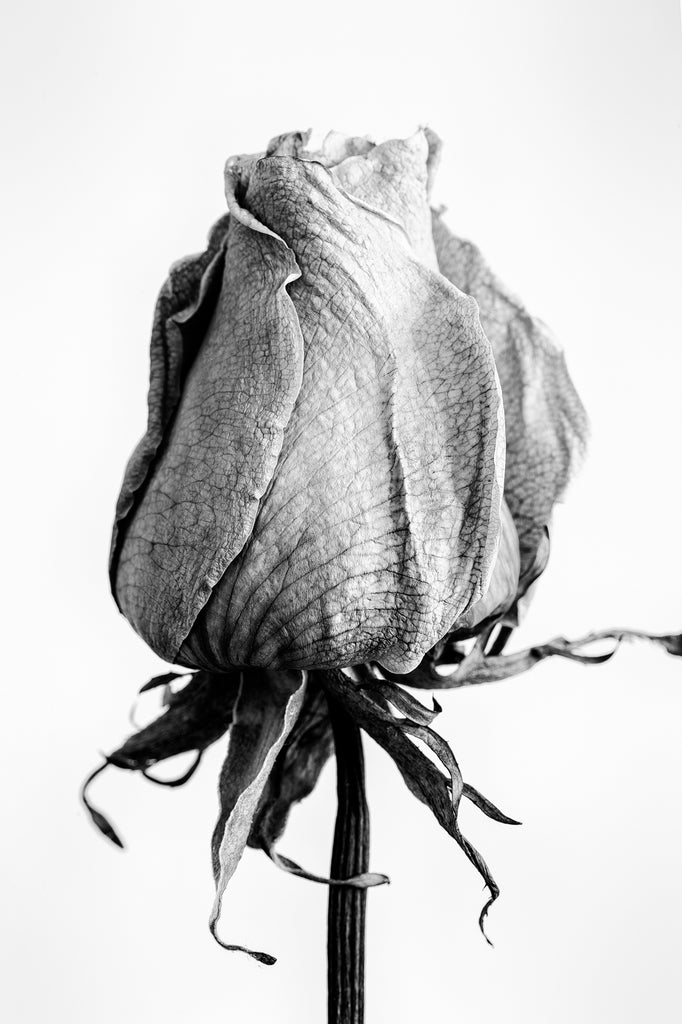This black and white photograph captures a close-up of a dying rose bud against a pure white background. The stem extends from the bottom of the image upwards to the tightly closed and shrunken bud of the rose. The rose appears unhealthy, with its petals tightly bound and twisted, resembling a teacup without an opening. The petals exhibit a dry, cracking texture, emphasizing the flower's withered state. Beneath the bud, scraggly, crumpled leaves hang from the stem, also appearing dried and wavy. The intricate veins of the deteriorating petals and leaves stand out starkly due to the intense lighting, which casts dramatic shadows and highlights. The withered beauty of the rose is heightened by the pure white backdrop, making the desiccated details of the flower's decline all the more poignant.